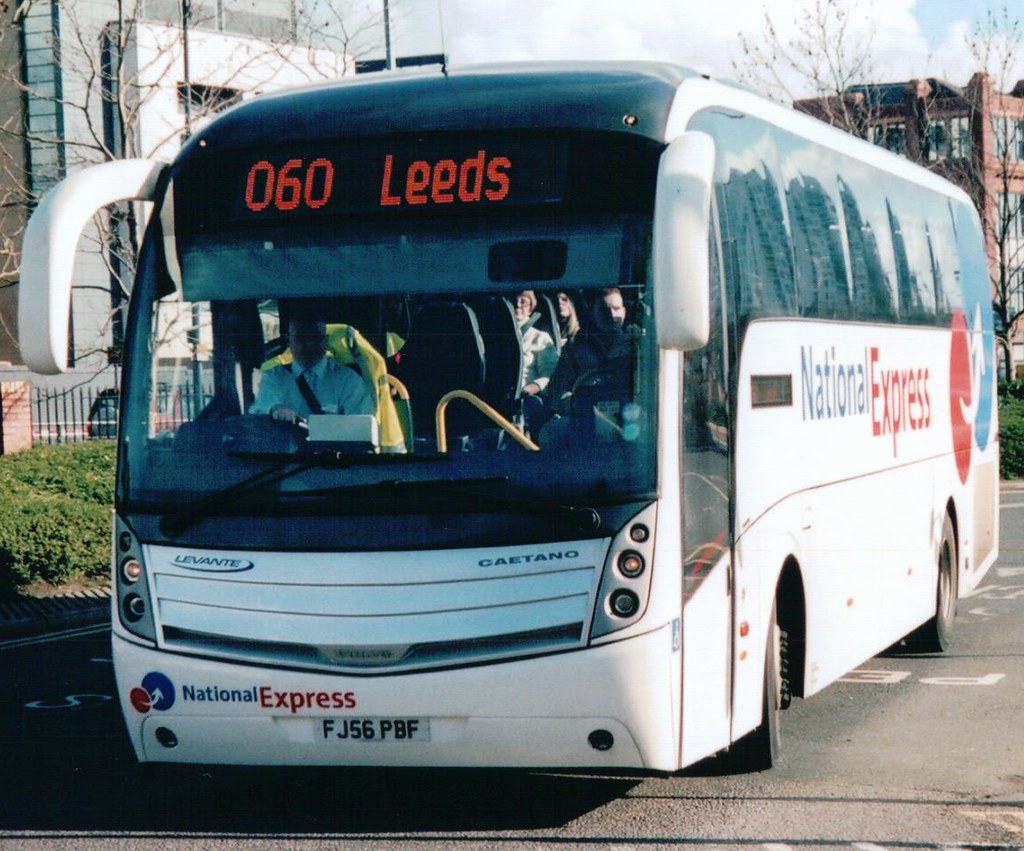The image depicts a modern white National Express bus, prominently featuring blue and red branding on the sides and front. The bus is facing the camera, showcasing its front and driver's side, with "060 Leeds" displayed in electronic orange letters at the top, signaling its destination. The driver, wearing a white shirt and seatbelt, is visible through the windshield, along with several passengers seated in the first few rows. The license plate reads FJ56PBF in black letters on a white background. 

The bus is positioned on a paved road, which has white lines and a blacktop surface. Surrounding the scene, you can see a mix of buildings—on the right, a red brick structure, and on the far left, a white building with lighter brown bricks. There are green bushes near the buildings, a black fence affixed to orange brick posts, and bare brown trees indicating a potentially chilly time of year. Above, the sky is partly cloudy, with patches of blue and fluffy white clouds. Despite the grainy and blurry quality of the photograph, these details frame the bus as it prepares to turn towards the camera.